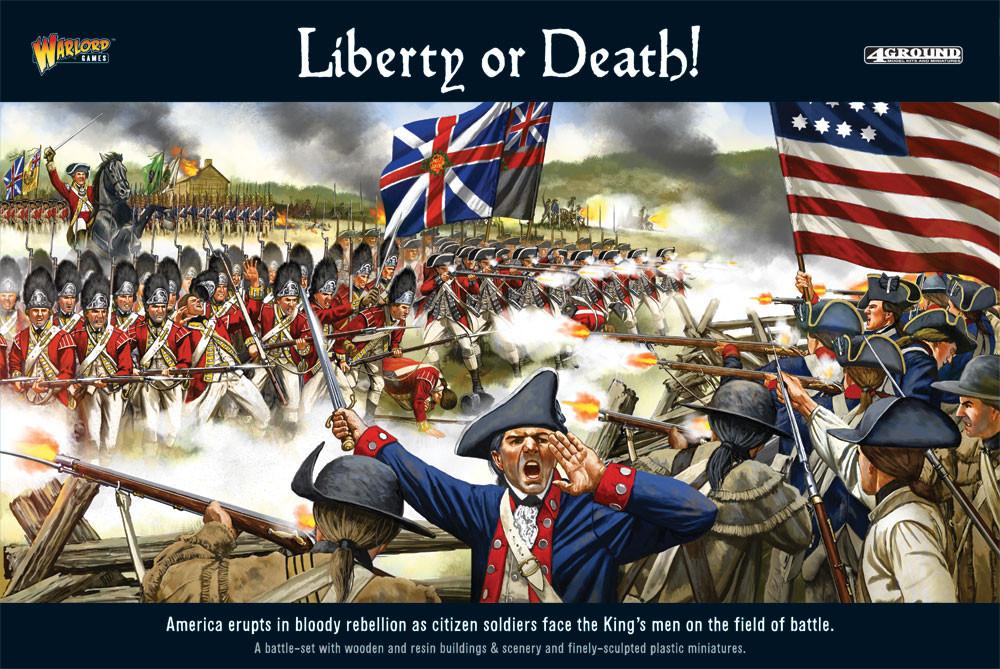This detailed illustration, titled "Liberty or Death," depicts a dramatic battle scene from the American Revolutionary War and is presented by Warlord Games with Foreground support. The image is framed by dark blue horizontal banners; the top banner reads "Liberty or Death," while the bottom one states, "America erupts in bloody rebellion as citizen-soldiers face the king's men on the field of battle, a battle set with wooden and resin buildings and scenery and finely sculpted plastic miniatures."

In the center of the image, British troops, known as Redcoats, are seen on the left, adorned in their iconic red uniforms with gold outlines, white sashes, and tall, furry blue hats with silver fronts. They carry the Union Jack and are armed with bayoneted muskets aimed towards the American forces. A British officer riding a rearing black horse leads them, his saber raised high, while behind him, a soldier holds the British flag.

On the right side, the American forces, clad in blue and gray uniforms with black hats, stand ready. An American officer, characterized by his blue coat with red stripes, white sash, black tricorn hat, and a long sword raised aloft, shouts commands. The American soldiers, some in uniform and others in militia or wilderness attire, fire back, their muskets discharging trails of smoke. Notably, one of the Americans holds a large flag featuring the 13 stars arranged in rows.

In the background, green hills and a cabin set ablaze with billowing black smoke create a dramatic backdrop under a clear blue sky. Scattered across the battlefield are fallen British soldiers, emphasizing the chaos and carnage of war. The entire scene captures the intense conflict typical of miniature war games, enhanced by the detailed scenery and fine craftsmanship of the figures and setting.